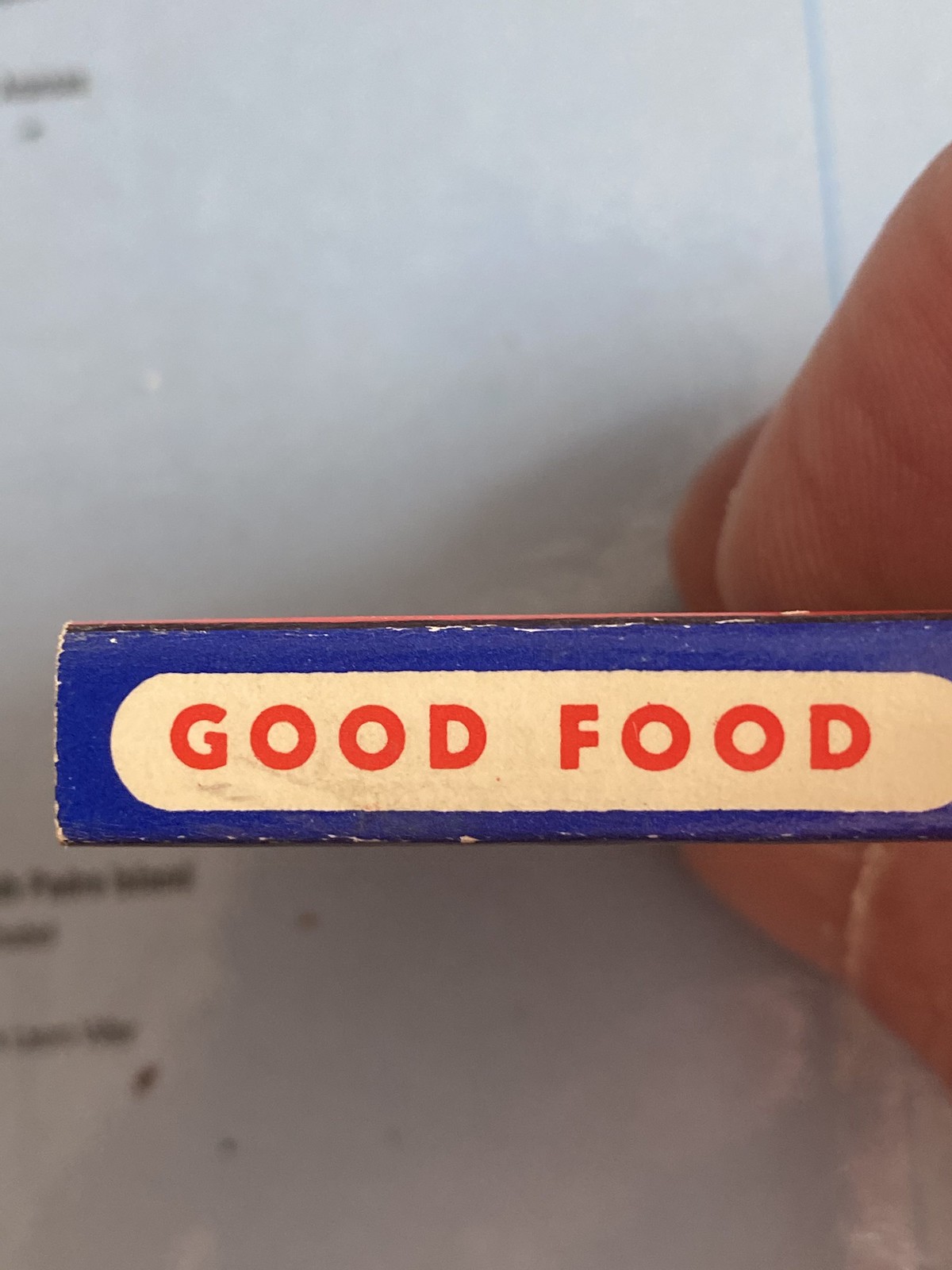This is a detailed, color photograph of a person's right hand holding a small, rectangular object, likely resembling the shape of a deck of cards. The person’s thumb and two fingers are clearly visible, pinching the object from either side. The object itself is blue, adorned with a white oval in the center, within which bold, red capital letters spell out "GOOD FOOD." This item is positioned on a flat, white sheet of paper, which has some black text on it that is out of focus and unreadable. The image provides a downward perspective, capturing the vivid details of both the object and the person’s grip.